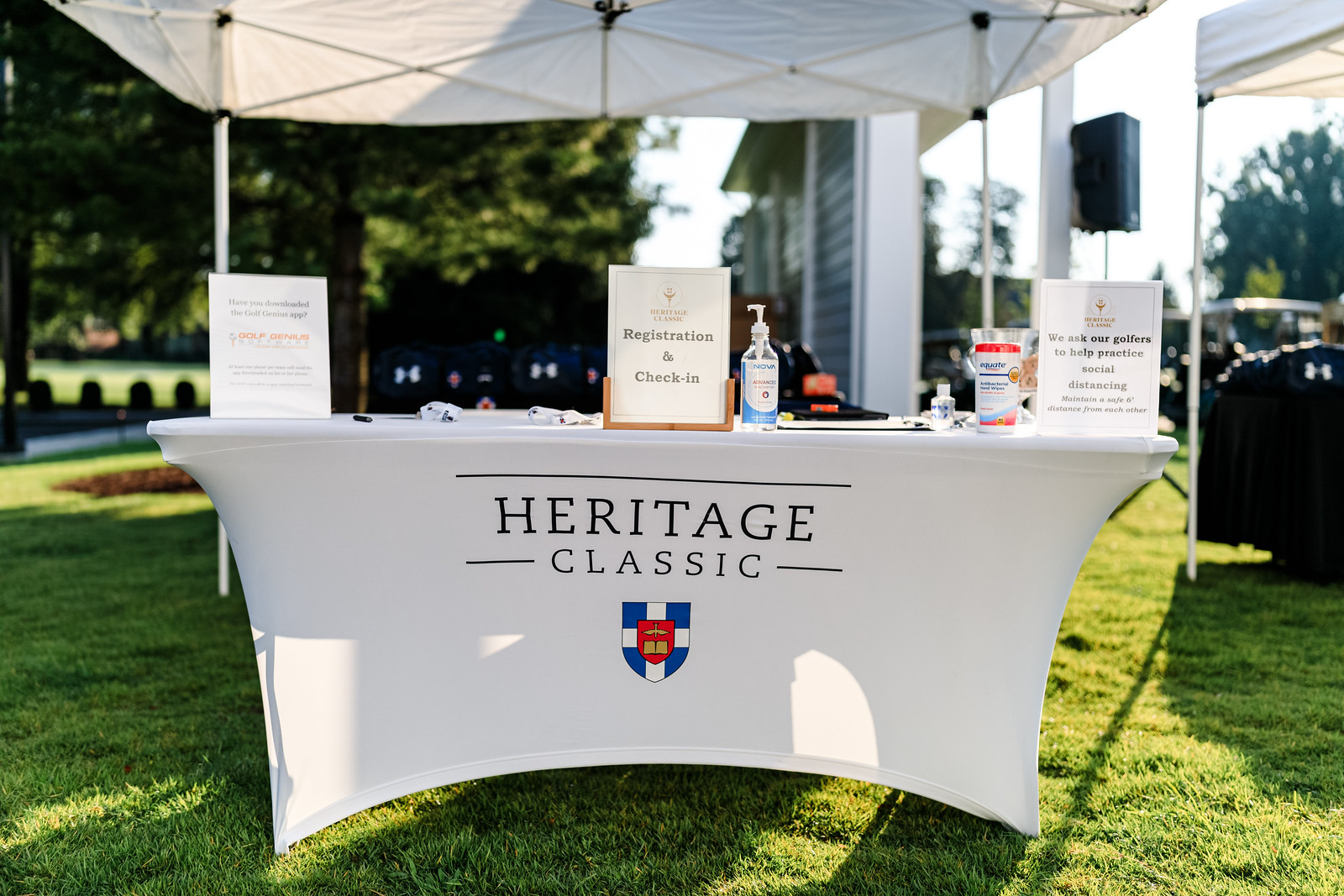This image captures an outdoor setup likely at a golf course, featuring a green grass surface. Central to the scene is a white table, draped with a fabric cover that prominently displays "Heritage Classic" in black lettering. Below this text is a distinctive shield design incorporating blue, white, and red colors, with interior elements such as a check pattern, a book, and a bird.

The table is clearly designated for registration and check-in for the Heritage Classic golf tournament, as indicated by multiple signs propped up on it. One central sign explicitly states "Registration and Check-In," while another advises golfers to practice social distancing, stating, "We ask our golfers to help practice social distancing." A third sign promotes downloading the Golf Genius app.

On the tabletop, several items are neatly arranged, including a pump bottle of hand sanitizer, wipes, a clipboard, pens, and lanyards, suggesting health precautions are being observed, likely due to COVID-19.

The background features several elements such as pop-up tents, trees, a visible sky, and a divided wall area. The absence of people suggests that the registration area is either not yet open or temporarily unattended. Overall, this detailed scene sets the stage for the start of the Heritage Classic golf event.